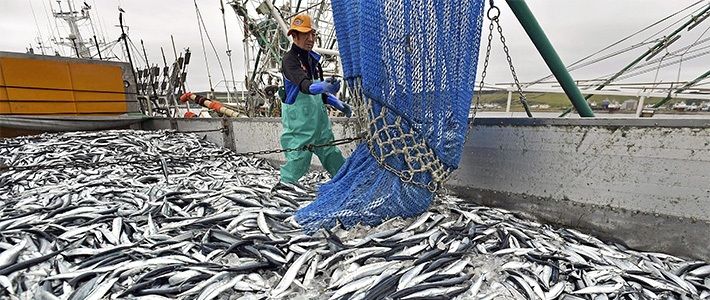In the photograph, a man stands at the center of a large, metallic gray fishing vessel, actively engaged in commercial fishing. He wears a yellow cap tilted sideways, blue gloves, and light blue or mint-green overalls. He is in the process of emptying a massive blue industrial net, from which countless fish are pouring out onto the ship's deck. The fish are densely packed, possibly numbering in the thousands, and are primarily gray and black, appearing dead and measuring around 8 to 10 inches in length. Behind the man, there is a yellow and gray square structure, likely an access point to the ship, and in the background, hints of water and a green hill can be seen, further emphasizing the maritime setting.